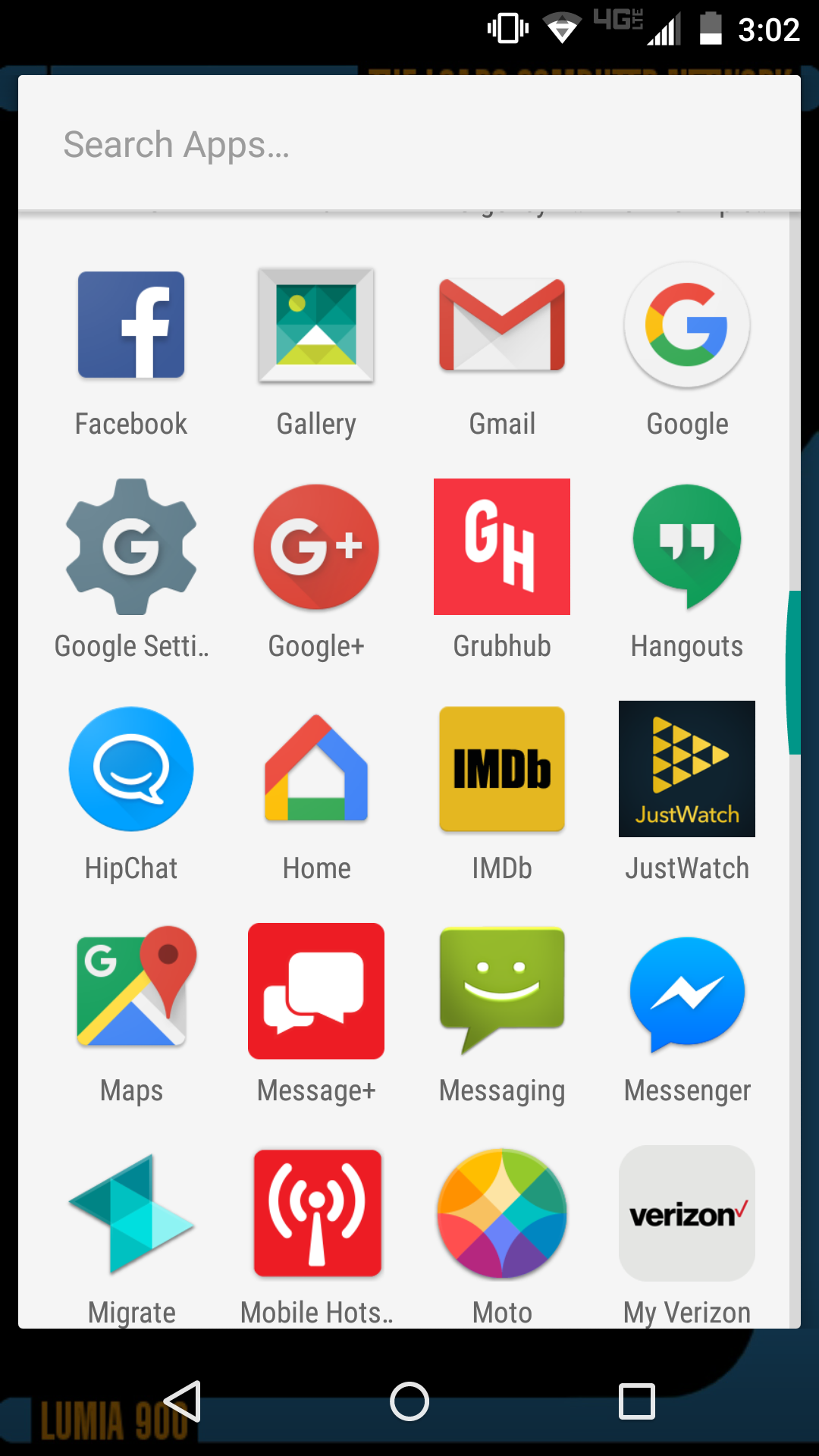The image depicts a neatly organized grid layout of 20 app icons on an Android device's app menu, presented in 5 rows of 4 icons each. The classic design of the icons suggests the image is from an older Android version. Recognizable apps include a variety of Google services such as Google, Gmail, Google Home, Google Maps, and the obsolete Google+. Legacy icons such as the old Messaging app and a bygone Facebook icon further hint at the image's age. Other apps visible in the image include Gallery, Grubhub, Hangouts, HipChat, IMDB, Just Watch, Message+, Messenger, Migrate, Mobile Hotspot, Moto, and My Verizon. The screen displays the time as 3:02, without specifying AM or PM, and features a search bar labeled "Search apps." The overall background is plain white, typical of a phone's menu screen, and there are no additional subtle details beyond the grid-format arrangement and the alphabetical sorting of app names.